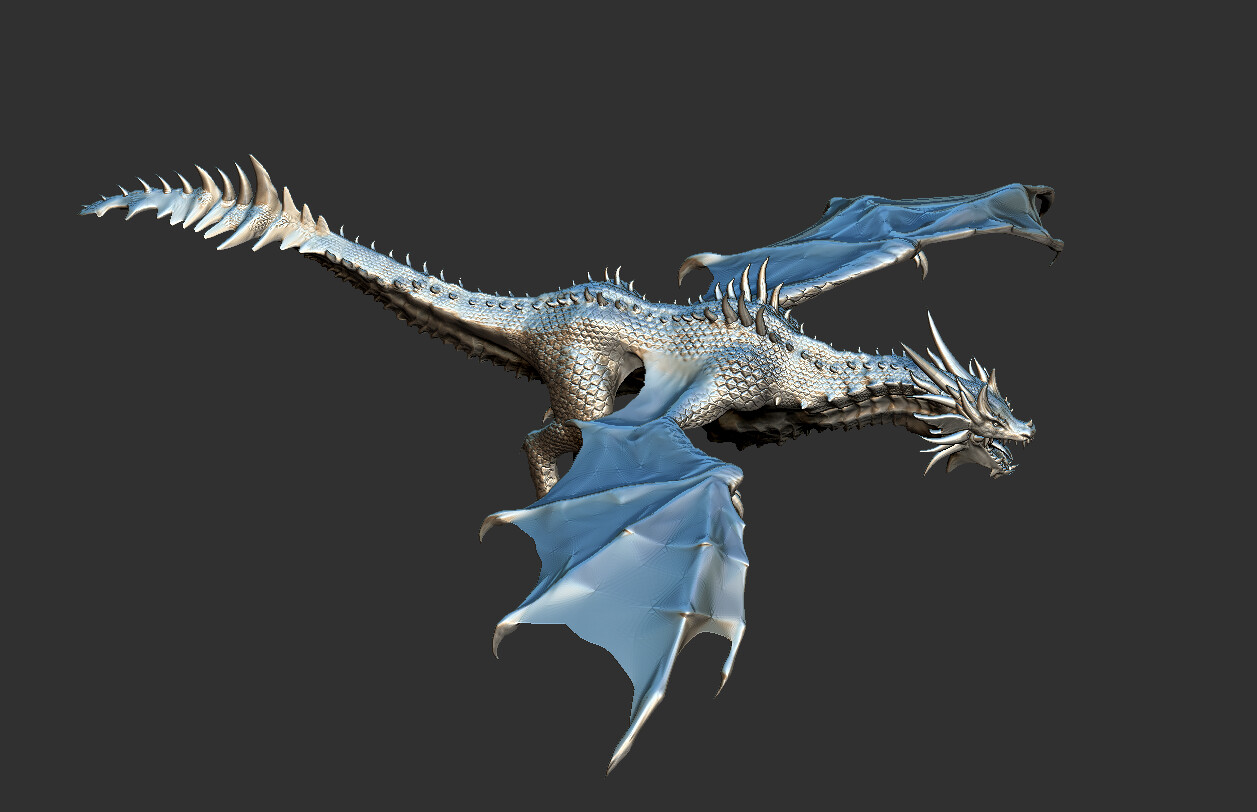This digital 3D rendering captures a magnificent, mythical dragon in mid-flight, showcasing its awe-inspiring form against a dark gray background. The dragon, covered entirely in silver scales, exhibits two large, robust hind legs and outstretched wings replacing where arms would normally be. The wings, smooth in texture yet ending in formidable talons, add to its menacing grace. The lizard-like head, open to reveal sharp fangs, is adorned with a crown of multiple talons and horns forming an impressive crest. These horns extend from its head down its back to the very tip of its long, spike-riddled tail, contributing to its fierce and majestic appearance. The image emphasizes the dragon's metallic sheen, which enhances its otherworldly presence.